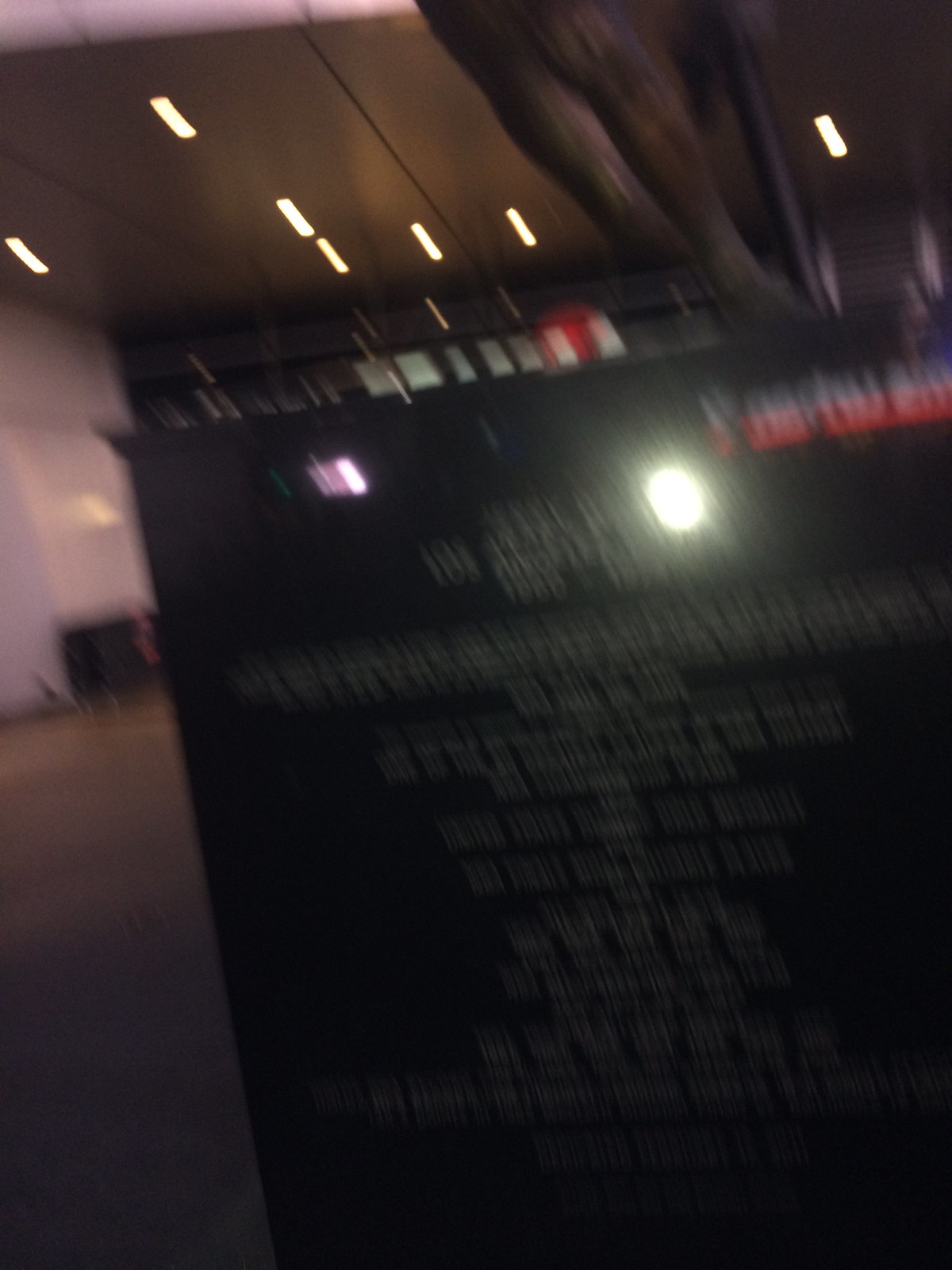This indoor photograph suffers from low light conditions, resulting in a slow shutter speed that causes noticeable motion blur, likely due to camera movement. In the foreground, there's a piece of machinery featuring a light at its top. Although the writing on the side of the machinery is obscured by the blur, it appears to be in white. The background reveals an open space with a visible ceiling and wall, both also affected by the blur. Additional lights in the distance are equally blurred, emphasizing the overall lack of sharpness in the image.